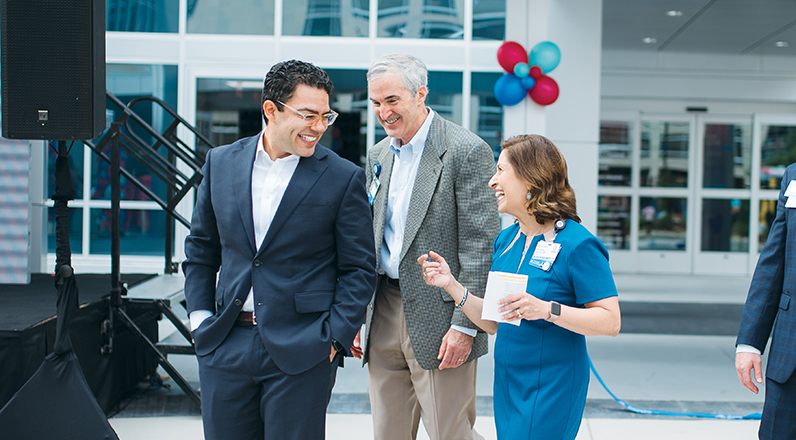In this vibrant photo, three individuals are captured in sharp focus against a slightly blurred backdrop of a white building adorned with numerous windows. The building features an indented section revealing an automatic door. To the left, just in view, is the corner of a black stage, accompanied by a speaker mounted on a pole and what appears to be a staircase leading up to the stage.

The trio at the center of the frame are all smiling, exuding an air of happiness and camaraderie. On the left, a man in a well-fitted blue suit and glasses grins warmly. Next to him, an older gentleman with gray hair sports a gray suit jacket over a white shirt and tan pants, his suit jacket open and casual. He and the woman to his left both wear badges, possibly indicating their roles at an event or within an organization. The woman, with her brown hair and elegant blue dress, accessorizes with a smartwatch and completes the group with her friendly expression.

In the periphery of the photograph, to the right, the arm of another individual in a blue suit is faintly visible. Brightening the scene, bunches of blue and red balloons are strategically attached to the building, adding a festive touch to the setting.